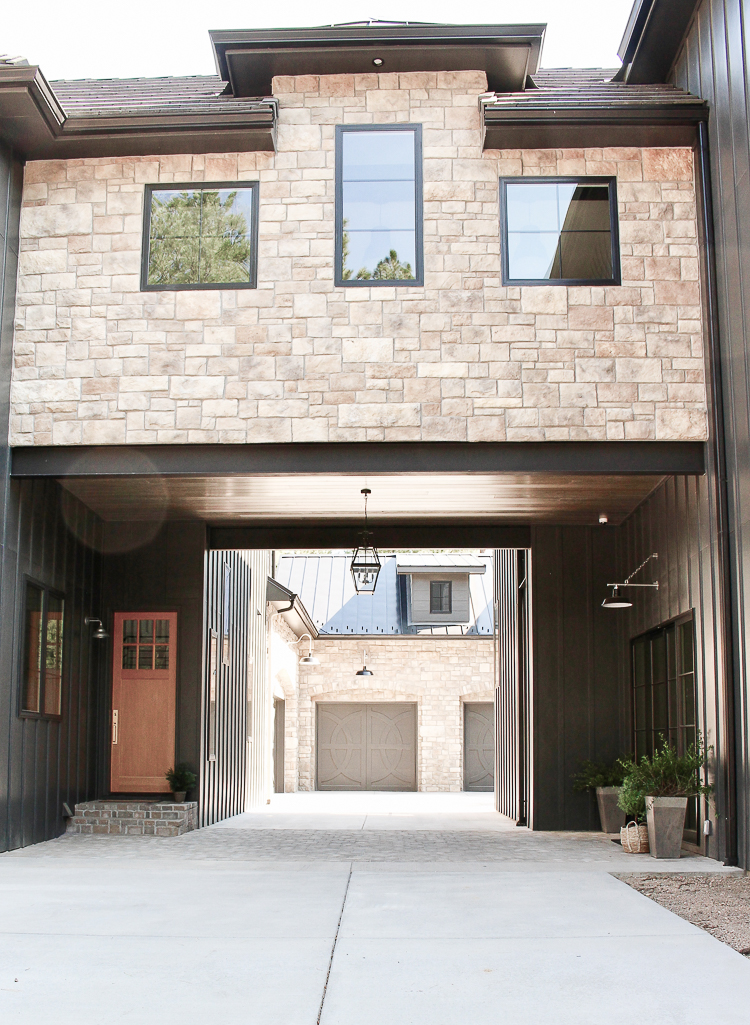This photograph captures the exterior of a large building, potentially an apartment complex or a grand house, featuring an arched driveway that leads into an inner courtyard. The driveway is constructed of bright concrete with stonework accents near the doors. The archway, composed of various shades of pale brown and tan stones, includes three windows and stretches over the driveway, suggesting it might house living quarters above. To the left, there is an unassuming wooden door for pedestrian access, while at the end of the driveway, there are garage doors for vehicles. Additional details include a lamp hanging from the ceiling of the overhang, potted plants along the right side, and various other doors and windows enhancing the structure's façade. The photograph, taken on a bright, sunlit day, reveals more of the building's roofline and other architectural features.